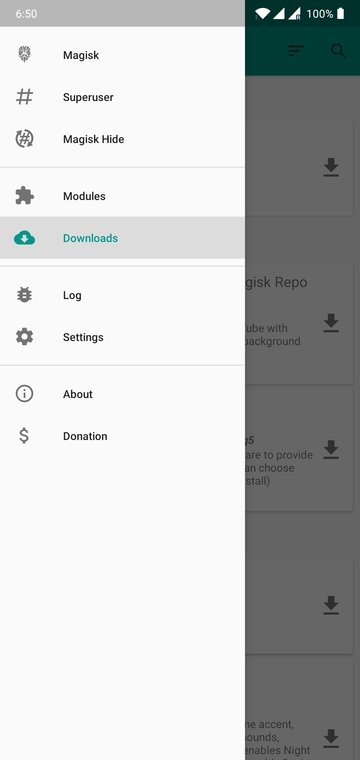This image captures the screen interface of a mobile device showcasing the Magisk application. The timestamp displayed in the top left corner reads "6:50". On the top right corner, there are several status icons including cellular signal strength, WiFi connectivity, and battery status, which indicates a full charge at 100%.

On the left side of the screen, a vertical sidebar presents several tabs, each accompanied by an icon. These tabs, listed from top to bottom, are as follows:
- "Magisk" (M-A-G-I-S-K)
- "Super User"
- "Magisk Hide"
- "Modules"
- "Downloads" (depicted with a cloud icon)
- "Log" (represented by a bug icon)
- "Settings" (illustrated with a gear icon)
- "About" (symbolized with an information 'i' icon)
- "Donations" (depicted with a money symbol icon)

Each tab serves a unique function within the Magisk app, enhancing device management and customization.